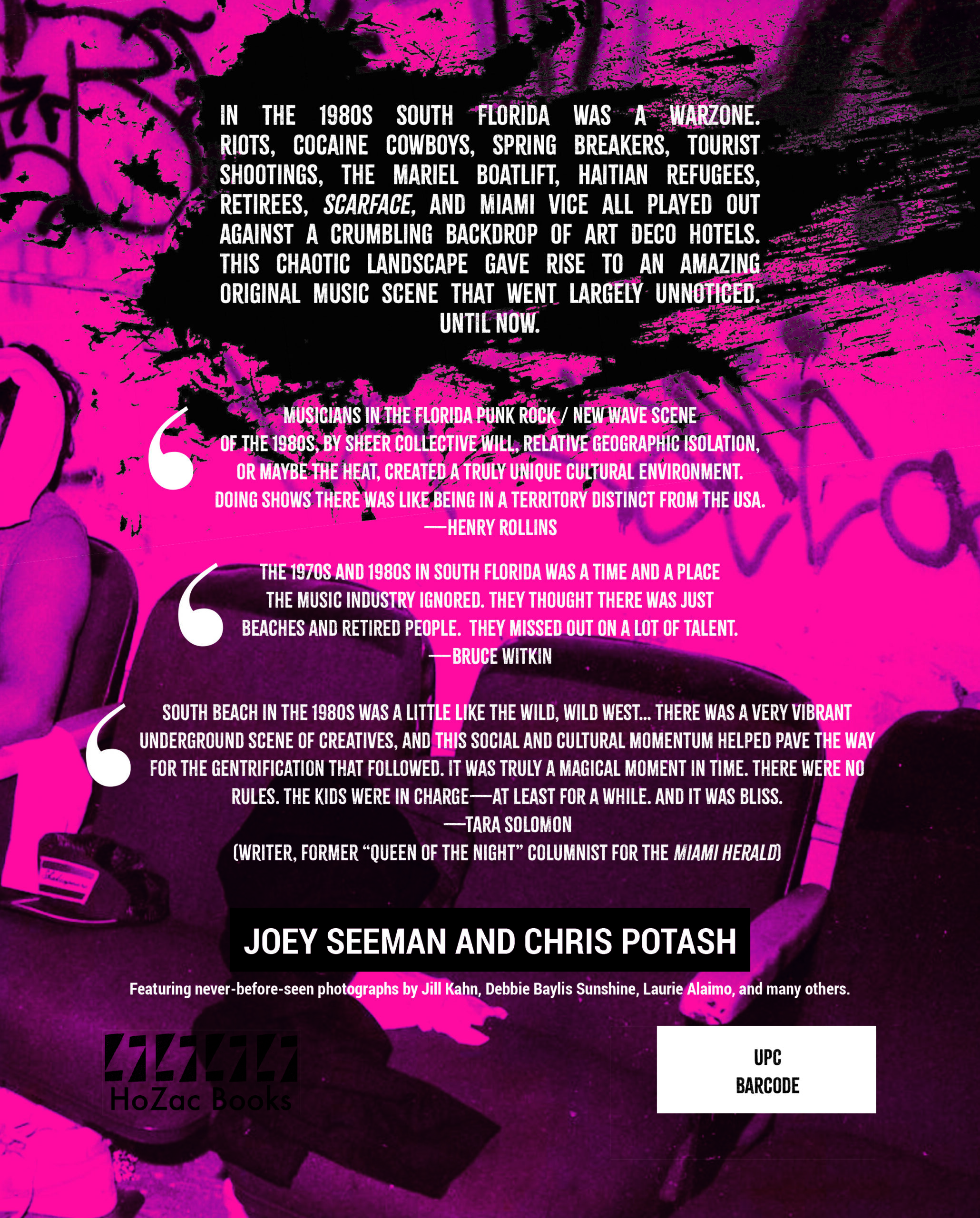The image features a vibrant, graffiti-themed poster with a bright pink and black background, adorned with various blocks of text over faded, graffiti-styled seat rows. The text chronicles the turbulent and dynamic history of South Florida during the 1980s, describing it as a "war zone" rife with riots, cocaine cowboys, spring breakers, tourist shootings, the Mariel Boatlift, Haitian refugees, retirees, Scarface, and Miami Vice. All these dramatic events unfolded against a crumbling backdrop of Art Deco hotels. This chaotic environment fostered a unique music scene in South Florida, particularly an overlooked and original punk rock and new wave scene. The isolation and intense heat contributed to its distinct cultural flavor. Crediting this vibrant underground culture are quotes from Henry Rollins, Bruce Witkin, and Tara Solomon, who recall South Beach in the 1980s as a ‘wild, wild West’ and a magical moment in time where the kids ruled. Featured in the text are Joey Seaman and Chris Potash, with contributions from photographers like Jill Kahn, Debbie Bayless-Sunshine, and Lori Alaimo, among others. The bottom of the image includes a white box with a UPC barcode and mentions Hozak Books.